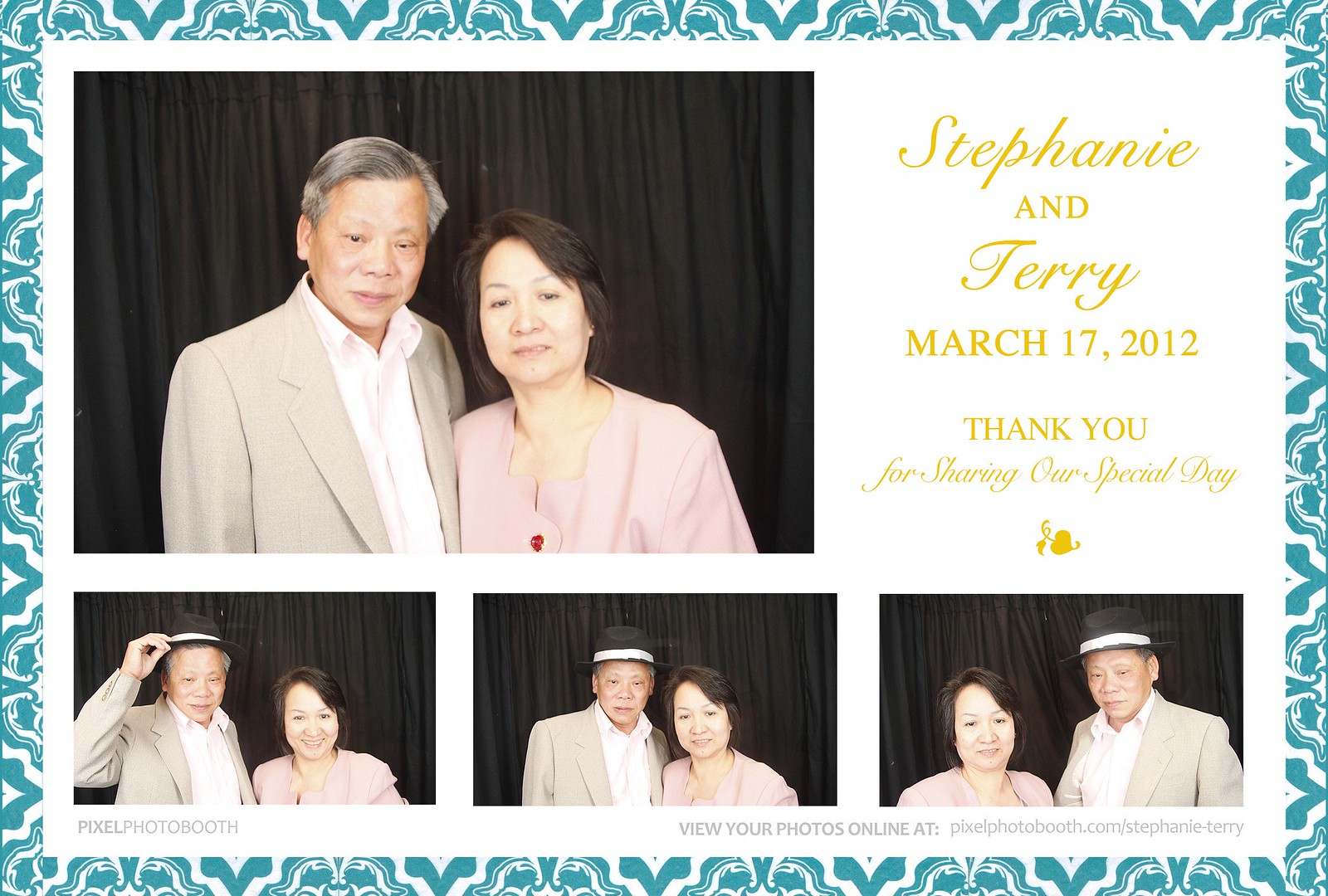On the left side of the rectangular card, there is a notice for a Saint Patrick's Day wedding featuring elegant gold lettering. The names "Stephanie" and "Terry" are written with a slant to the right, and the date "March 17, 2012" is in normal print. It also says, "Thank you for sharing our special day" in a decorative print with a small gold icon underneath.

The inside of the card has a white background bordered by a green sculpted design. Prominently featured is a large photograph of an Asian couple against a black backdrop in the top left. The man, older with gray hair and wearing a tan suit coat and white dress shirt, stands to the left of the woman who has black hair and wears a pink dress. Both have serious expressions. Below this main picture are three smaller photos: one shows the man touching his hat with a playful expression, the center photo depicts the woman smiling, and the far-right picture shows the couple in a loving pose with switched positions; she is now on the left and he on the right.

The upper right of the card repeats the names "Stephanie and Terry, March 17, 2012," in yellow letters. Below the photos, in light gray print hard to read, it says "Pixel Photo Booth. View your photos online at..."